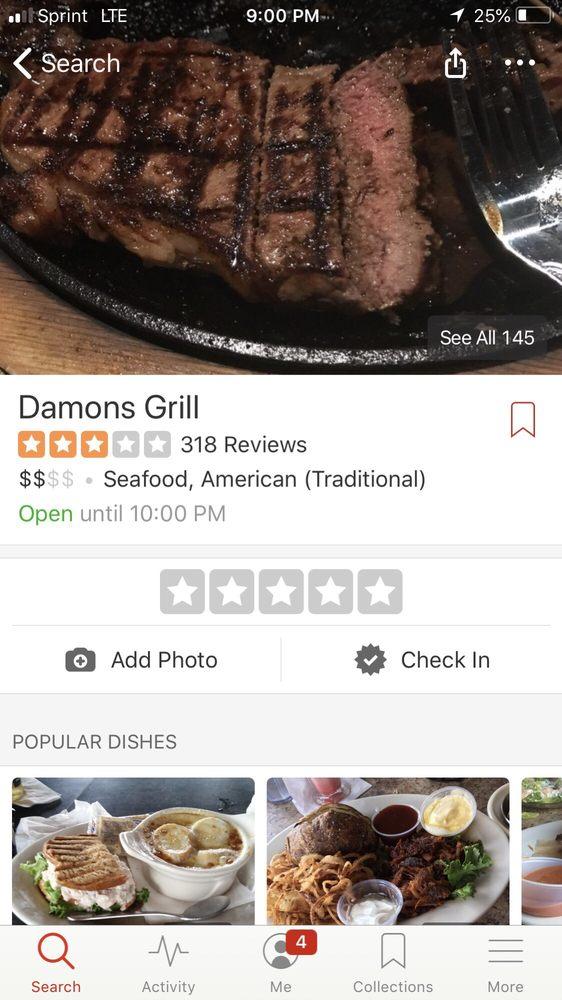The image depicts a mobile screen displaying the Yelp app open to a restaurant's page. The top section of the screen indicates that the user is in the "Me" tab, with a badge labeled "Fulbright" signaling an unread notification. The restaurant featured is Damon's Grill, rated 3 out of 5 stars based on 318 reviews, and categorized under seafood and traditional American cuisine with a moderate price range ($$).

At the center of the screen is an appetizing photograph of a medium-cooked steak, cut in the middle to reveal its juicy interior. Forks are placed nearby, enhancing the visual appeal. Users are given the option to add their own rating, photos, or check in at the restaurant.

In the lower portion, the section "Popular Dishes" is displayed, featuring images of various meals. One dish appears to be a perfectly grilled piece of chicken, while another includes fries paired with grilled shrimp, surrounded by Yelp's familiar user interface elements, predominantly white in the background.